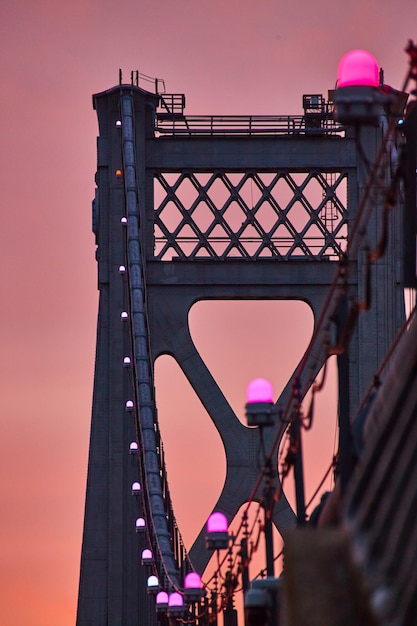The image showcases an unusual and artistic shot of the Golden Gate Bridge during dusk or dawn, under a dimly lit pink or mauve sky. Dominating the right side of the image is a strong close-up of a section of the bridge, featuring a series of upside-down dome-shaped lights lining the large cables. These lights start as dark pink in the foreground and transition to lighter pink, then ultimately to white, as they extend into the distance. One particular light, vividly detailed, is positioned in the upper right corner, seemingly at the top of the bridge. The image also reveals the bridge's distinctive architectural elements, including a tower and cross members forming a lattice or crisscross design between its pillars. The whole scene exudes an ethereal ambiance, enhanced by the unusual close-up perspective and the softly glowing illumination.